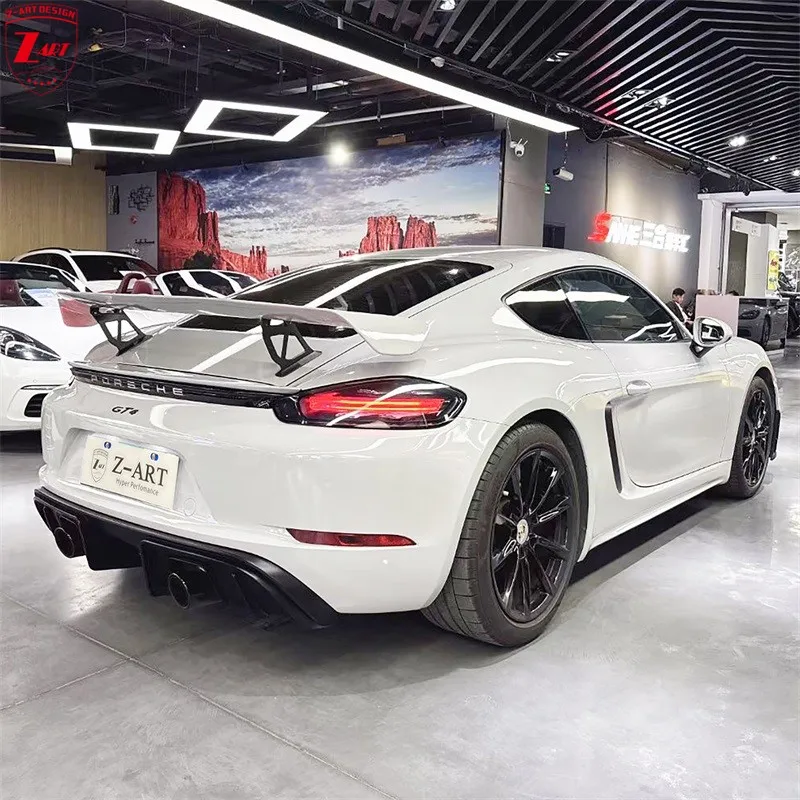This photograph captures a sleek, high-end car dealership showroom, prominently featuring a glossy white Porsche GT4 with a striking rear view. The car's distinctive features include a white spoiler, black tires and rims, and a special license plate reading "Z-ART" with the logo "GT4" and the brand "Porsche" displayed above it in elegant silver text. This modern, futuristic showroom is characterized by its industrial design, with a smudged gray concrete floor and a ridge of black beams supporting suspended lights, plus three diamond-shaped overhead lights enhancing the ambiance. 

To the far left, there is a pale wooden wall that adds a touch of warmth, while a vivid screen showcases a mural of a red rock canyon under a pale blue sky dotted with gray clouds, suggesting a Southwest desert landscape. Adjacent to this screen is an angled gray wall, accentuated by an LED sign featuring a mix of Latin and East Asian characters, though its exact message is indistinguishable from this angle.

In the background, there are glimpses of three more white sports cars with dark windshields, underscoring the dealership's premium collection. A desk with a person working on a computer indicates the business setting, along with a hard-to-read neon sign above the desk, potentially displaying 'S-N-I-E'. This meticulously detailed environment beautifully reflects the prestige and luxury associated with the showcased Porsche.